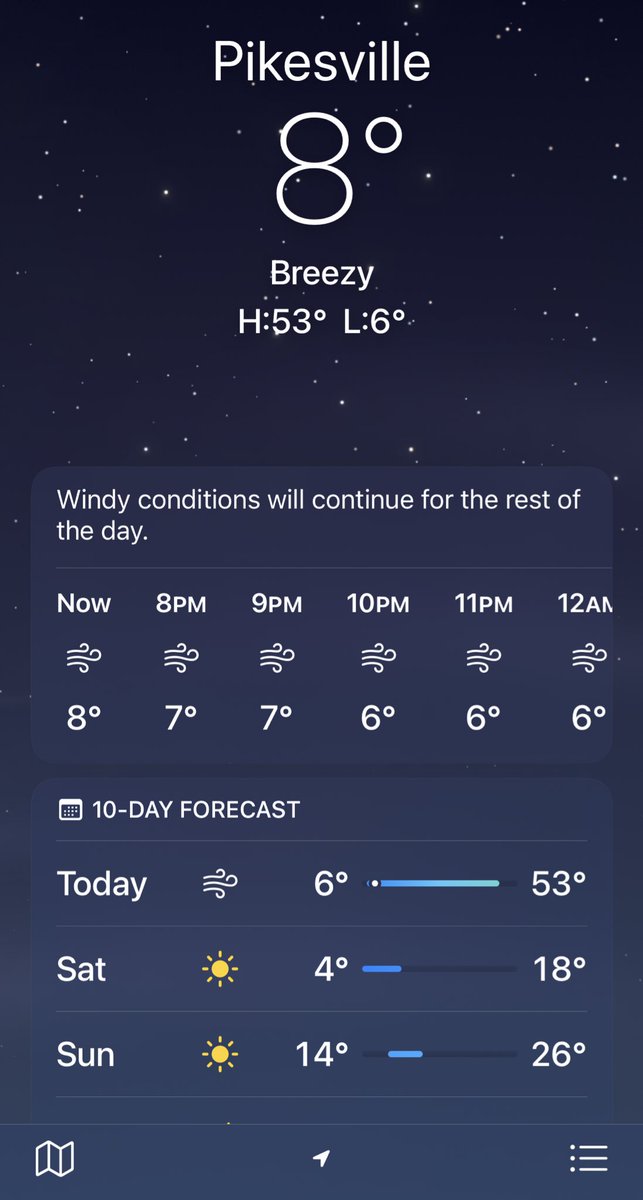The screenshot captures a mobile weather page with a night-time theme, highlighted by a dark blue background adorned with a starry sky. At the top center, the location is prominently displayed as "Pikesville" in large white text. Below it, the current temperature is shown as "8°" in large font, accompanied by the description "Breezy" and the day's high and low temperatures: "H: 53°, L: 6°."

The middle section of the screen is divided into two parts with a flat dark blue color. The first part states, "Windy conditions will continue for the rest of the day." The second part provides an hourly forecast from 8 p.m. to 12 a.m., indicating the following temperatures: 8°, 7°, 7°, 6°, and 6°. A wind icon accompanies these readings.

Below the hourly forecast, a "10-day forecast" box is displayed, marked by a calendar icon. It lists the weather for today, Saturday, and Sunday. Today, it will be windy with a temperature range from a low of 6° to a high of 53°. Saturday is expected to be sunny with a low of 4° and a high of 18°, while Sunday will also be sunny, ranging from 14° to 26°.

At the bottom of the image, two icons are positioned at the left and bottom corners, and a white arrow is centered in the footer.